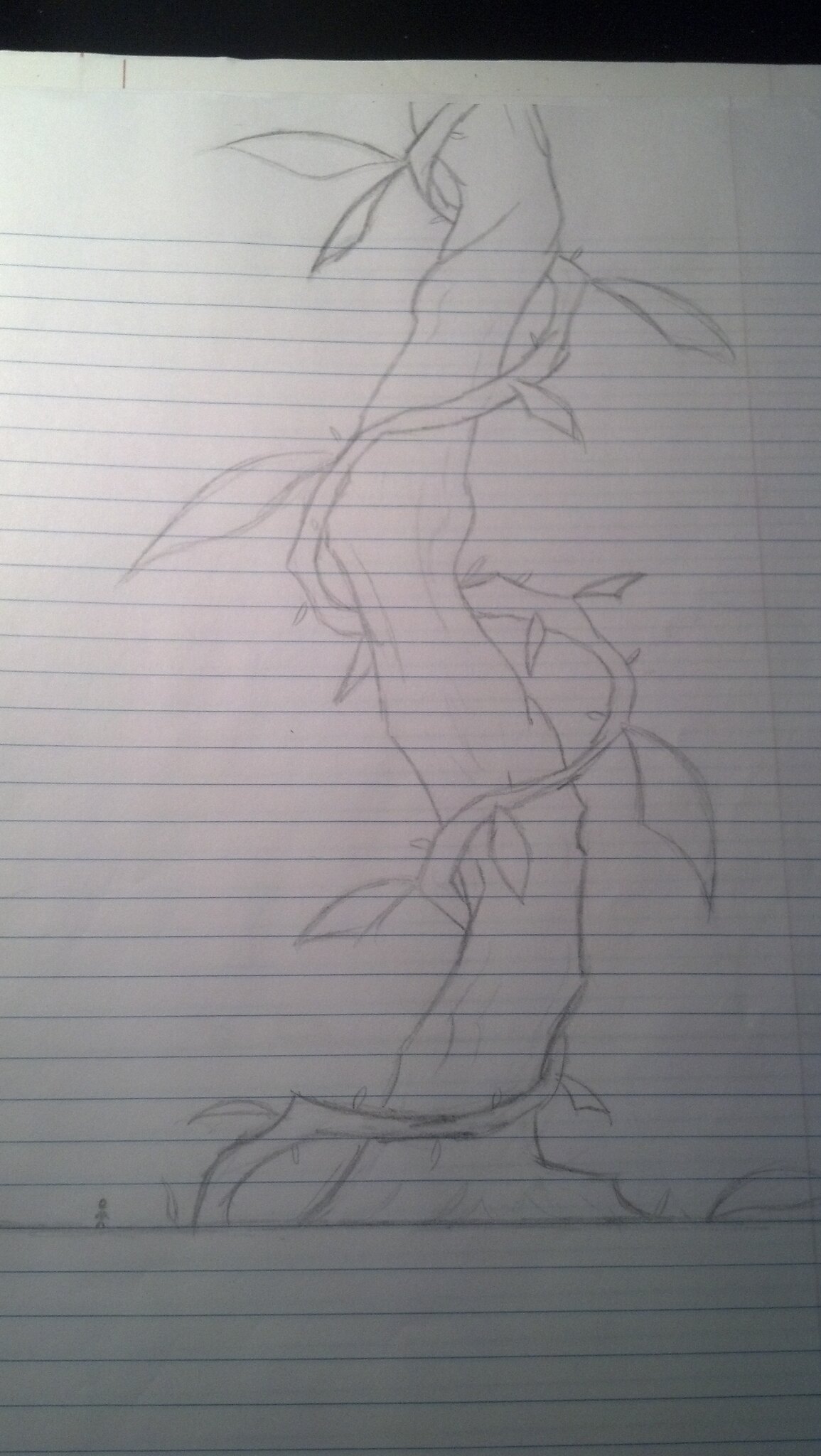The image is a detailed pencil drawing on notebook paper, capturing a sprawling, twisting tree with vines wrapped around it akin to a snake coiling around its prey. The tree starts at the pencil-drawn ground line at the bottom of the page and curves dramatically to the right, then left, then right again, creating an almost serpentine ascent. The giant vine begins at the top and spirals continuously down to the base, even penetrating the ground to the left. Small thorns and occasional leaves are illustrated along the vine, adding texture to the composition. The scale of the tree is emphasized by a tiny stick figure at the bottom left, who barely reaches a fraction of the tree's colossal height. The background features the edges of a black surface, indicating that the notebook paper rests on a table, with other sheets partially visible behind it, suggesting it might still be part of a notebook.